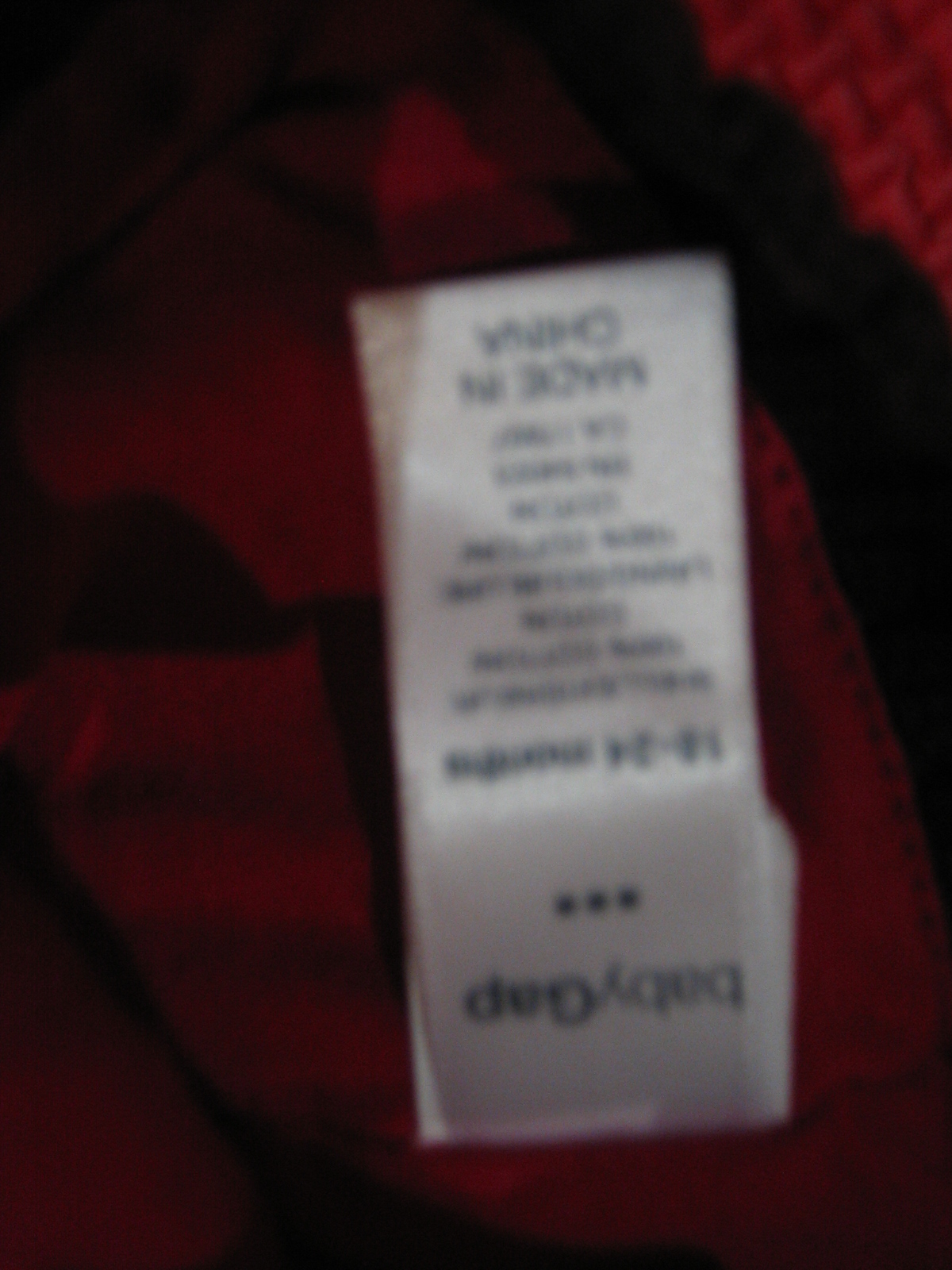This vertically oriented, color photograph captures an upside-down view of a fabric label from a Baby Gap item. The image appears blurred, making the text difficult to decipher. Despite the blur and inversion, the tag is recognizable as part of a red garment with visible black stitching, likely situated at a corner seam or along the inside collar. The label prominently features the Baby Gap logo with three dots beneath it, as well as size information indicating "12 to 24 months." Additional text, providing a description of the item, is also present but not entirely legible. At the bottom of the tag, in large black letters, is the phrase "Made in China." All elements in the image are presented upside down, and the overall scene is characterized by its lack of sharpness.